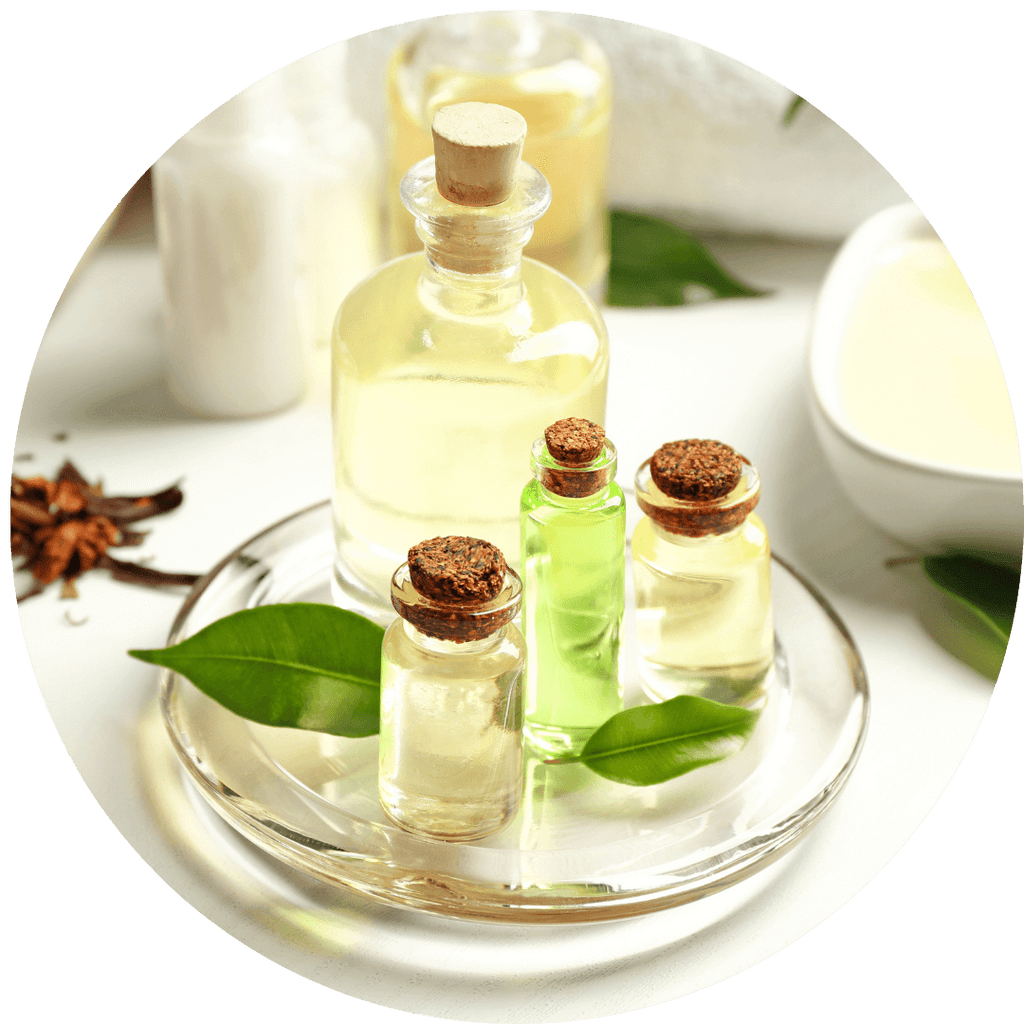The photograph, encased within a circular frame against a solid white background, showcases a carefully arranged scene on a flat white surface. In the center, a clear round glass plate holds an assortment of vials and a flask, each sealed with cork stoppers. Three small vials contain a yellowish clear liquid, while one taller, slender vial, located towards the middle, is filled with a light green liquid. Alongside the vials, two green leaves are artfully placed on the plate, offering a touch of nature. A larger flask, also with a cork stopper, is part of this arrangement, positioned towards the back. The background reveals more apothecary-style glass containers, some containing white and beige substances, and possibly a crumpled brown plant to the left. On the right side, a ceramic white bowl holds an ivory-colored liquid, accompanied by another green leaf in front of it. The entire composition evokes a serene and meticulously crafted natural laboratory setting.